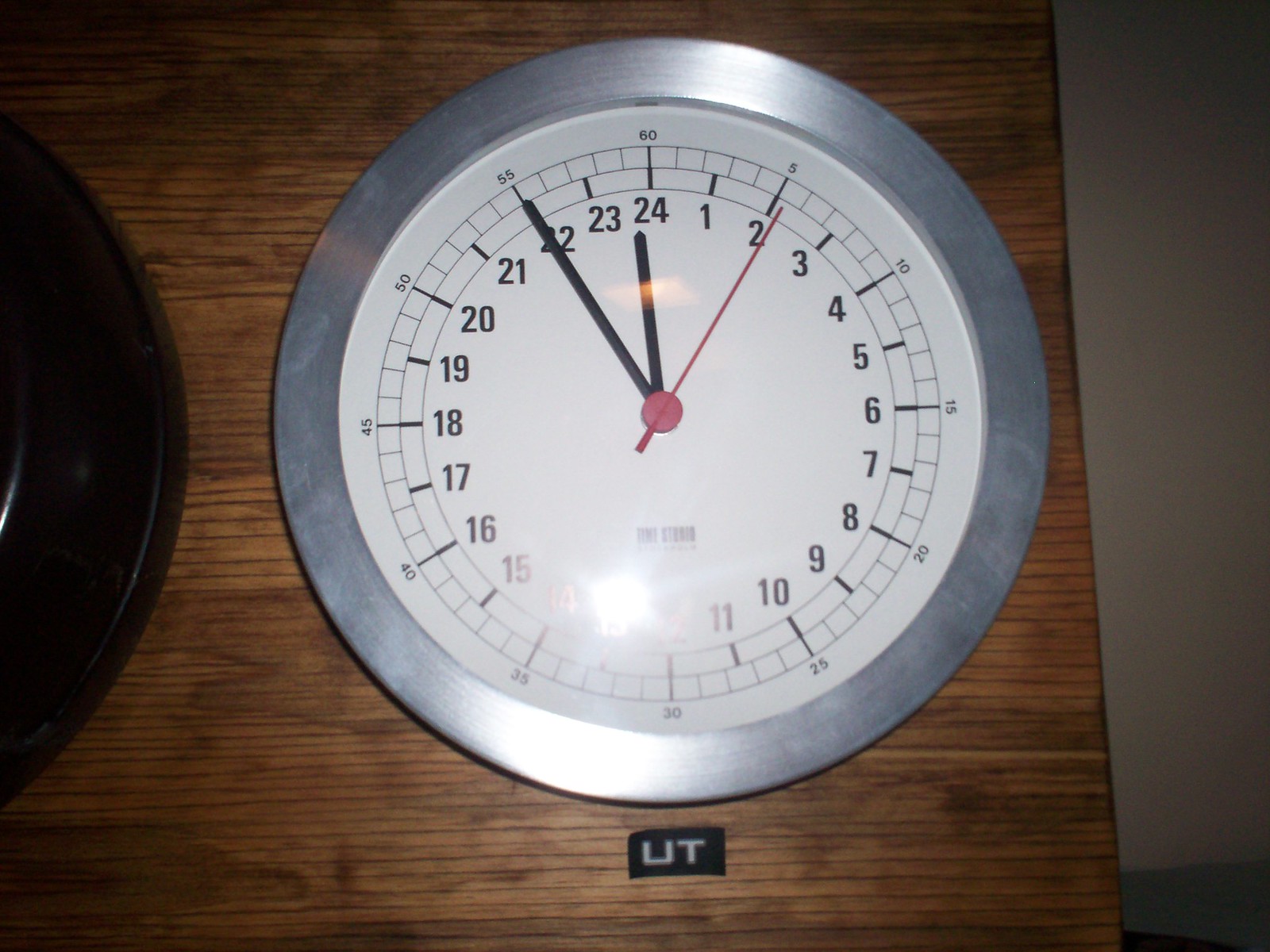A silver-rimmed, military-style clock is prominently displayed against a backdrop of dark brown, paneled wood. The clock's face, which is white, features a meticulous three-circle design. The outermost circle counts the minutes in groups of five, clearly marked from 5 to 60. Small boxes between each number further aid in precise time reading. The middle circle enhances the minute-hand movement with bold lines that extend inward, intersecting both the outer and middle rings. The innermost circle marks the hours in a 24-hour format, rather than the standard 12-hour setup. This detailed timepiece shows that it is currently 10 minutes before midnight, with the hour hand on the 24-hour mark and the minute hand on the 50-minute mark. Below the clock face, a small black box is labeled "UT", completing the clock's utilitarian appearance.